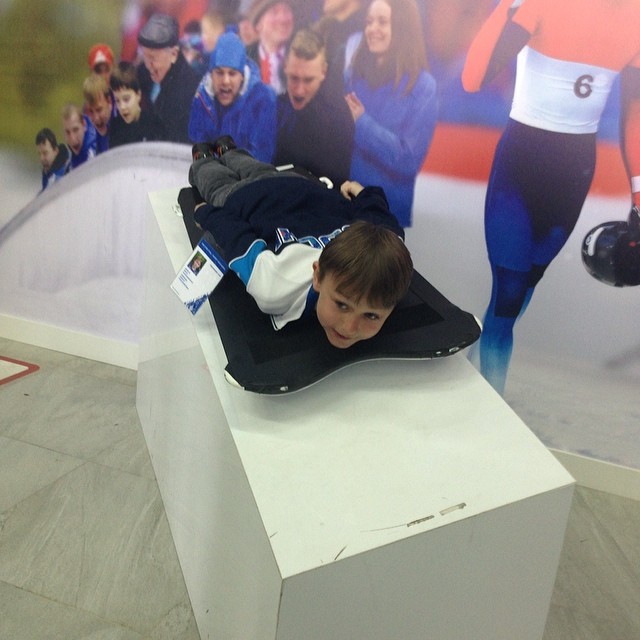This indoor photograph, cropped into a close-up, features a young boy, possibly around 5 or 6 years old, lying face down on a black sled atop a white rectangular pedestal, poised at the beginning of a steep, white slide. The boy, who has straight brown hair and dark eyes, wears gray pants and a navy blue, powder blue, and white long-sleeved jacket. His arms are neatly placed at his sides as he looks apprehensive. The floor beneath the pedestal is light gray stone tile. In the background, there is a poster featuring a crowd of people dressed in red, white, and blue, suggesting a cheering audience. Additionally, there is a partial image of an athlete clad in a skin-tight bodysuit with a reddish-orange top, white stripe across the torso bearing a black number six, and blue pants, holding a helmet. This gives the setting a competitive atmosphere, reminiscent of a tobogganing contest.